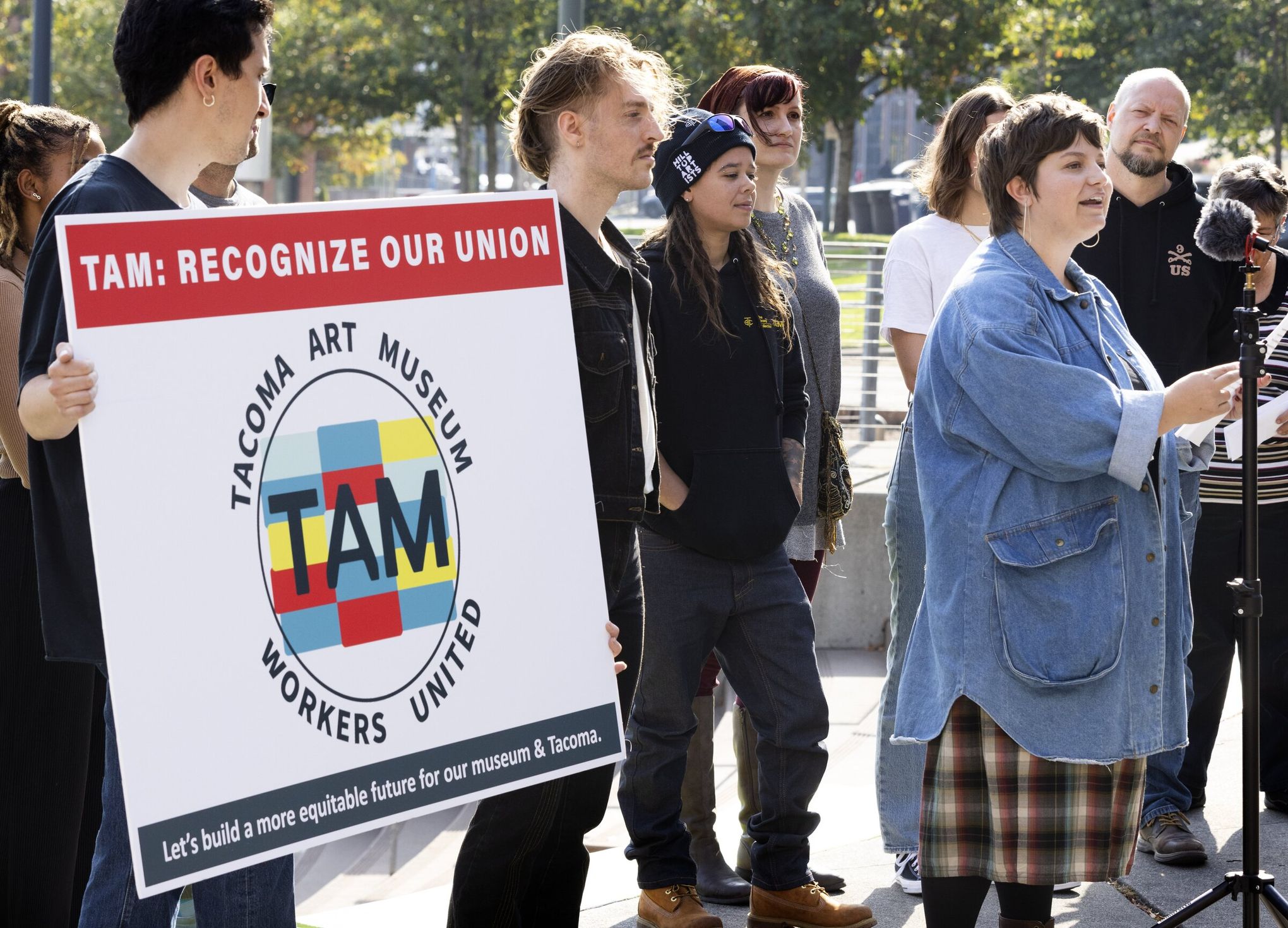This photograph captures a group of approximately nine adults standing outside on a concrete surface, beneath a backdrop of green trees and city scenery. The group, all facing the same direction, appears to be part of a gathering advocating for union recognition at the Tacoma Art Museum. Dominating the image is a woman with short brown hair, large hoop earrings, a denim shirt, and a plaid skirt, who stands prominently at a microphone with her mouth open, indicating she is speaking. She holds a piece of paper while addressing the group. To her left, another participant holds a large, detailed sign that reads, "T.A.M. Recognize Our Union" alongside a multicolored logo encircled by "Tacoma Art Museum Workers United," with the further message, "Let's build a more equitable future for our museum and Tacoma." The attendees, many of whom are wearing black, are lined up, somewhat informally, directly behind the speaker, with concrete, fencing, and lush green trees framing the scene.